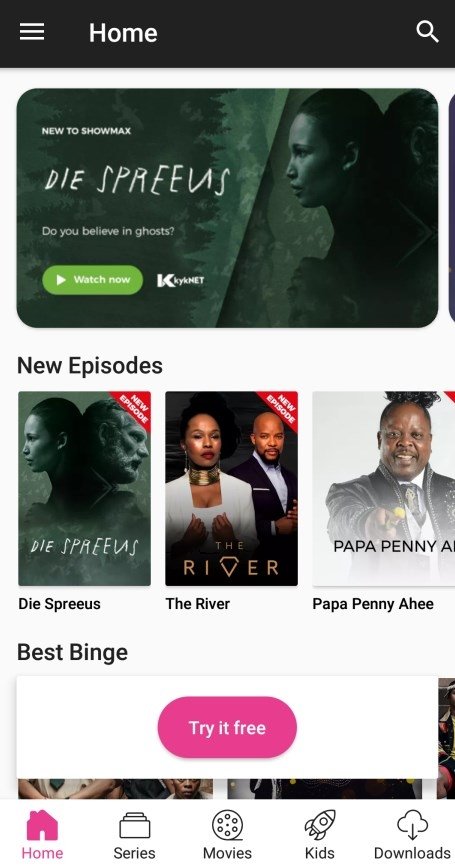The screenshot depicts the interface of a mobile phone displaying the homepage of a movie and TV show streaming application, presumably ShowMax, due to the appearance of that name in the layout.

At the very top, there are partial elements of the device's interface that are cut off, making it impossible to identify the specific type of mobile device. The visible portion starts with the app's navigation bar, which includes a "Home" label on the left, indicating the current tab, and a three-lined menu icon for more options. On the right side of this bar is an unopened search icon.

Beneath the navigation bar is the main content area of the app. At the top of this section is a prominent thumbnail for a show titled "Die Screens," accompanied by a tagline reading "Do You Believe in Ghosts?" This thumbnail has a dark, monotone forest green hue and features an image of a young woman in a forest, viewed in side profile. Just below this thumbnail is a vibrant green "Watch Now" button. The top of the page also notes "New to ShowMax," which hints that this is a featured new release on the platform.

Following this section is a horizontal bar labeled "New Episodes," showcasing a scrolling reel of series thumbnails. Visible in the screenshot are three shows: "Die Spears," "The River," and "Papa Penny Ahi."

Further down, the next section is titled "Best Binge," though the specific thumbnails for this category are partially obscured by a bright pink button urging users to "Try It Free."

At the bottom of the interface, a navigation bar offers several options: "Home," "Series," "Movies," "Kids," and "Download," indicating the different sections users can explore within the app.